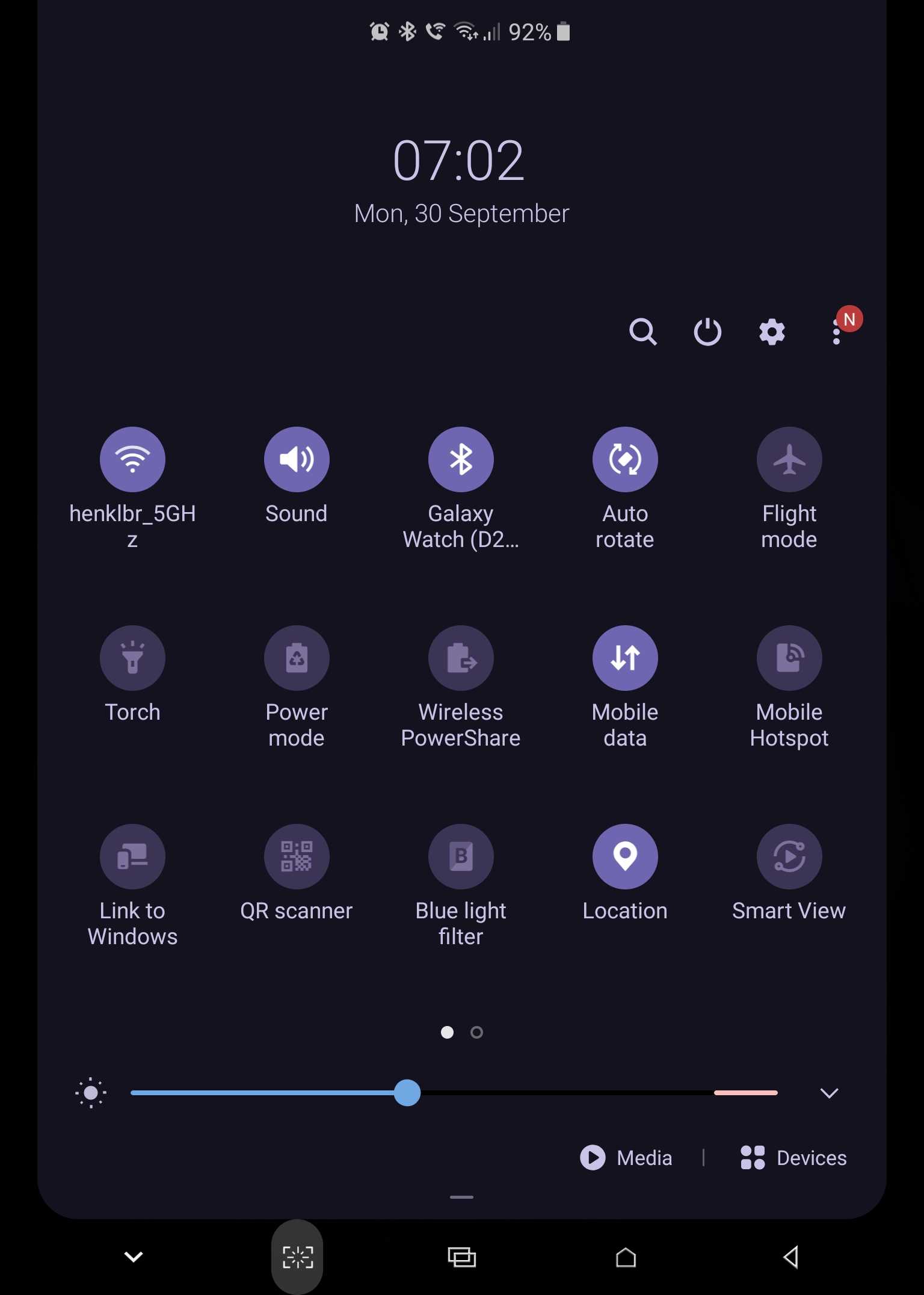Here is the cleaned-up and detailed caption for the image:

---

The image is a rectangular screenshot with the long side oriented vertically, seemingly captured from a tablet. At the very top, the status bar displays an array of icons: an alarm clock, Bluetooth symbol, phone icon, Wi-Fi connectivity, cellular connectivity, and a battery indicator showing 92% charge. The image is encased in a black border, which slightly blends with the very dark gray background at the center of the screen.

Directly below the status bar, the screen shows the time and date: "7:02," with "Monday, 30th of September" displayed underneath. Moving further down, slightly towards the right side, there are four primary control icons: a magnifying glass for search, a power icon, a settings gear icon, and an icon of three vertical dots with a red circle containing the letter "N," possibly indicating a notification.

Below these primary control icons, the remainder of the screen is occupied by a grid of 15 secondary icons arranged in a clean and organized layout. These icons represent various functions, listed in the following order: Wi-Fi, sound, Galaxy Watch, auto-rotate, flight mode, torch, power mode, wireless power share, mobile data, mobile hotspot, link to Windows, QR scanner, blue light filter, location services, and smart view.

This detailed layout of icons and information exemplifies the typical home screen arrangement for a tablet interface, providing quick access to essential functions and settings.